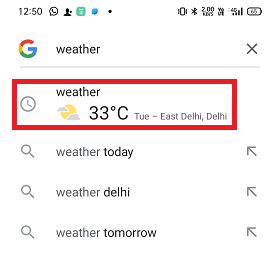This is a detailed screenshot of a mobile device's home screen, captured at 12:50 PM. At the top of the screen, the status bar features several icons. These include the time ("12:50"), a phone icon, a person icon, an unspecified green icon, and a smaller unrecognizable icon. To the right, there are the vibrate mode icon, the Bluetooth icon, another unrecognizable icon, the 4G network indicator with full signal bars, and the battery icon showing 65% charge remaining.

Below the status bar is a white search box housing the Google logo and a weather summary, with a gray "X" button for clearing the box. Immediately below this, a red-highlighted section displays a weather widget. This widget contains an image of a clock, a weather update showing a partly cloudy condition with a temperature of 33°C, and details such as "Tuesday" and "East Delhi."

Further down are three non-highlighted options for weather-related searches. These options include a search bar labeled "weather today" with an upward-facing arrow and a search icon, another labeled "weather in Delhi" with a similar arrow and search icon, and a third named "weather tomorrow" also with an arrow and search icon. The only actively selected and visible search result is the weather update for East Delhi, showing a temperature of 33°C.